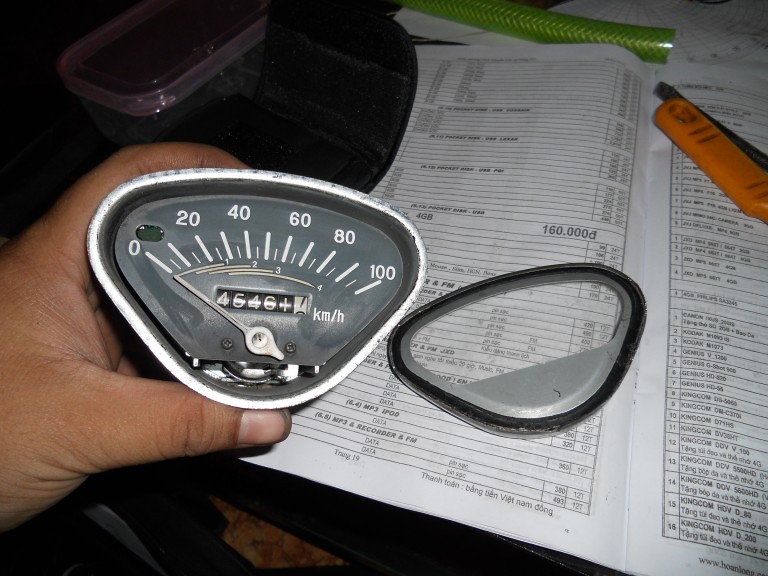This photo captures a handheld odometer displaying both miles and kilometers per hour. The velocity scale is marked with numbers 0, 20, 40, 80, and 100, indicating speed measurements. The odometer shows a reading of 4546 kilometers. The person holding the device has placed its clear plastic cover on top of a piece of paper. The paper underneath is filled with various numbers, names, and car parts information, and includes references to MP3, recorder, FM, and iPod. In the background, an orange box cutter, a neon green plastic object, and a Tupperware container are visible, adding context to the cluttered and busy setting.